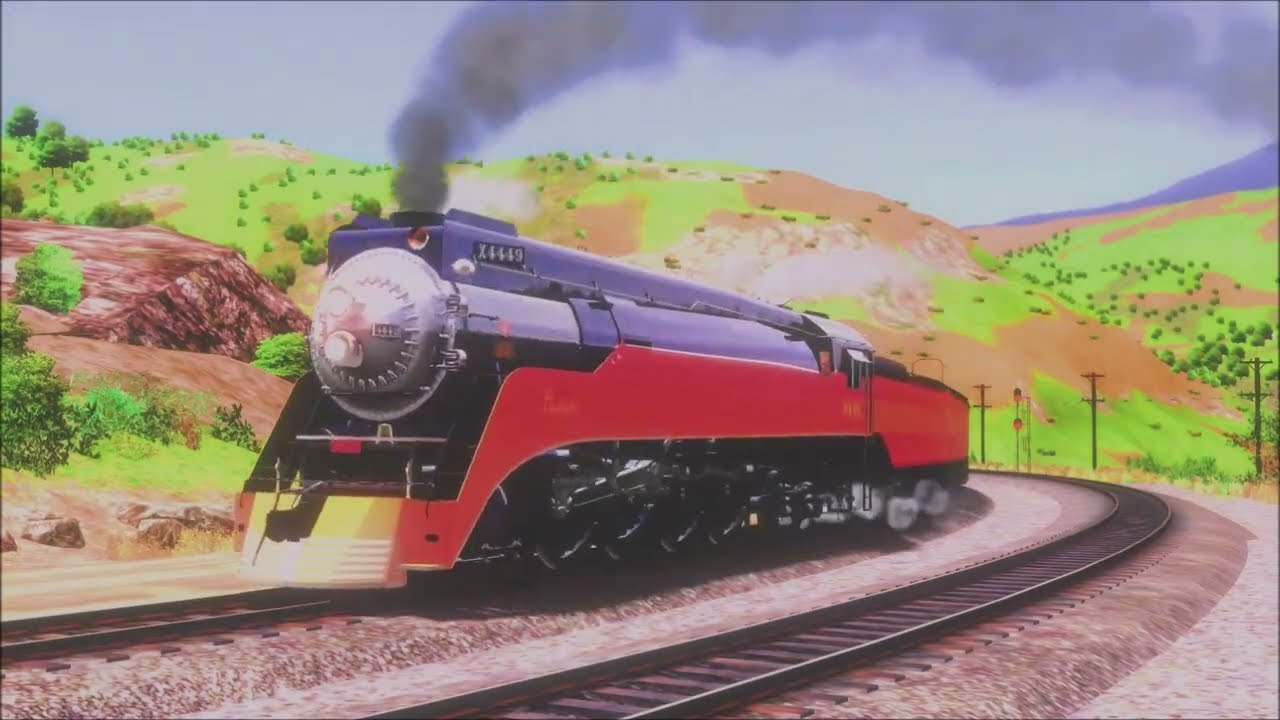The illustration depicts a sleek, narrow locomotive engine with a shiny silver round front end. The train features bright red sides, black wheels, and a bluish-colored top. Smoke billows from the top front of the engine, drifting upwards and towards the right-hand corner of the image. The locomotive is positioned on the right-hand set of two curved railroad tracks, facing outward and coming around a corner. An adjacent set of tracks remains empty. The scene is set in a rugged, rocky gravel landscape featuring a country hillside with vibrant green foliage and brownish rocks. Mountains with trees and a purple hue rise in the background, beneath a deep gray-blue sky. A line of telephone poles runs alongside the tracks, adding to the rural atmosphere.